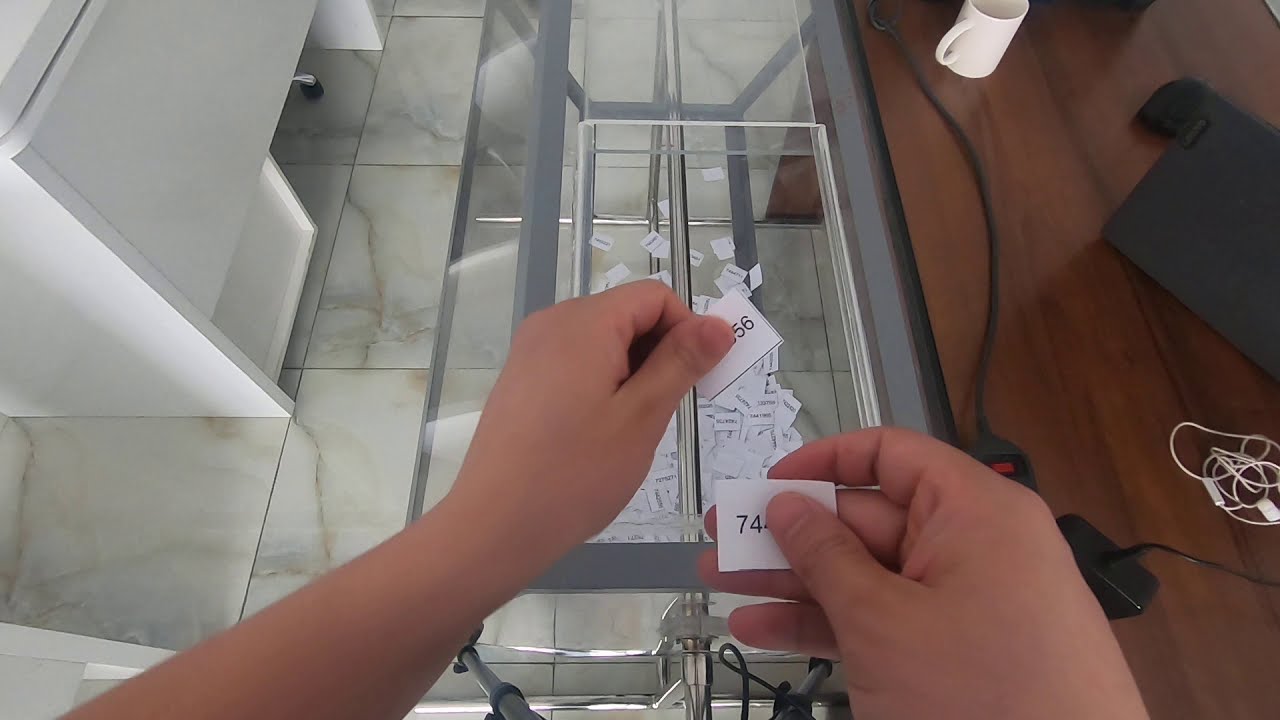The image captures a first-person view looking down at a scene where two hands are prominently featured, suggesting they belong to different individuals. The hands are interacting with a clear lucite box filled with small, rectangular pieces of white paper, each approximately an inch in size and labeled with black numbers. The right hand holds a piece of paper displaying the numbers "74," partly obscured by the thumb, while the left hand holds another paper showing the numbers "56." Surrounding the lucite box, the environment includes a wooden surface, likely a desk or table, with a coffee mug and some electrical cords on the right side. To the left, there's a section of a white desk, and the floor beneath and around the box is made of marble tiles with characteristic lines running through them.